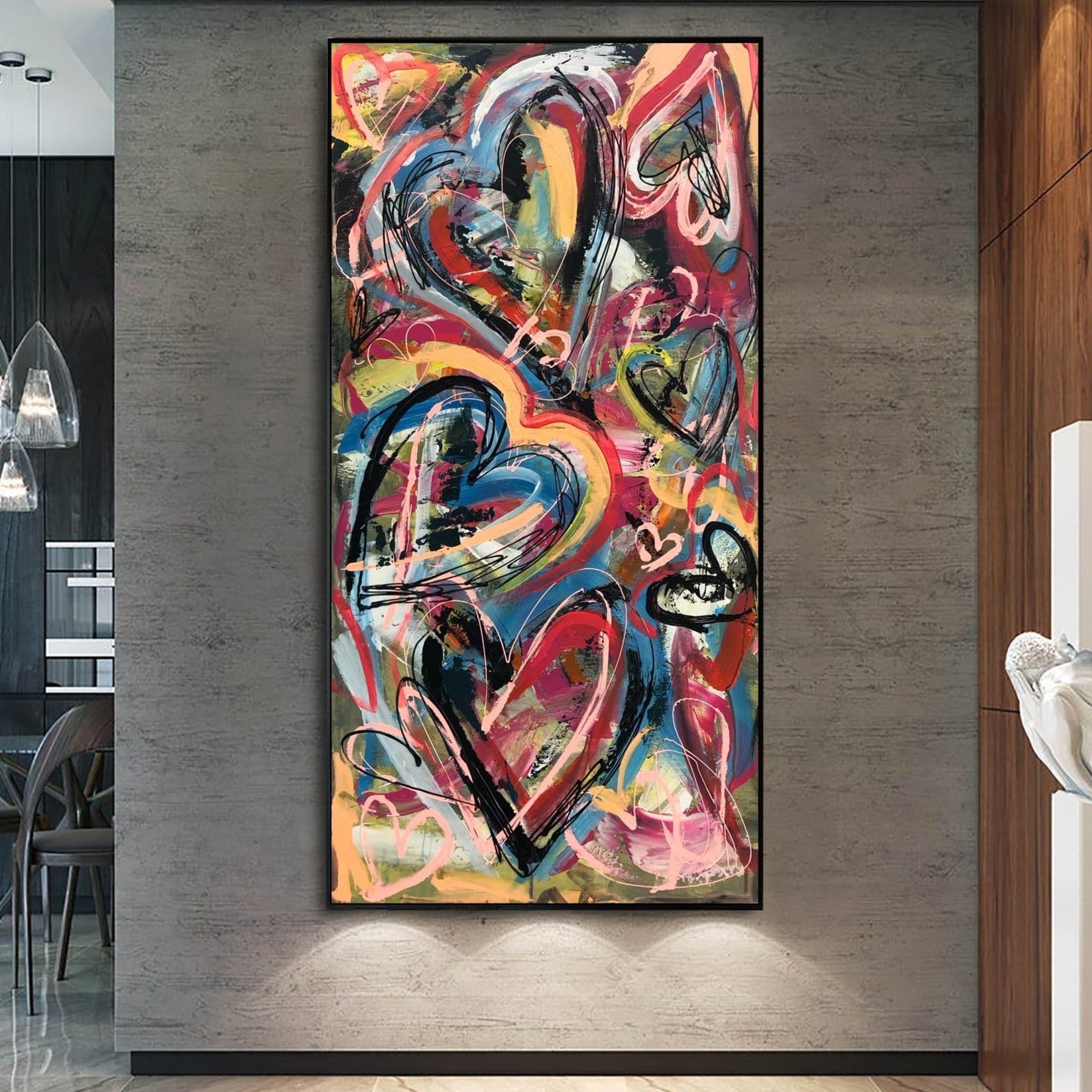The image features an almost illustration-style composition set against a stone-colored wall, predominantly gray. Central to the scene is an artwork with a slender black frame. This vibrant piece displays a collection of abstract hearts, each outlined in black and rendered using an array of vivid colors: olive green, yellow, white, lavender, pink, magenta, light blue, dark blue, green, lime green, gold, pale blue, red, and orange. Among these colorful hearts are some pale pink ones faintly outlined. To the left of the central image, there's a section of a mid-toned brown wooden wall and a partial view of a white sculpture. On the right, a glimpse of a table and a few gray chairs is visible, capped by a white overhead light fixture.